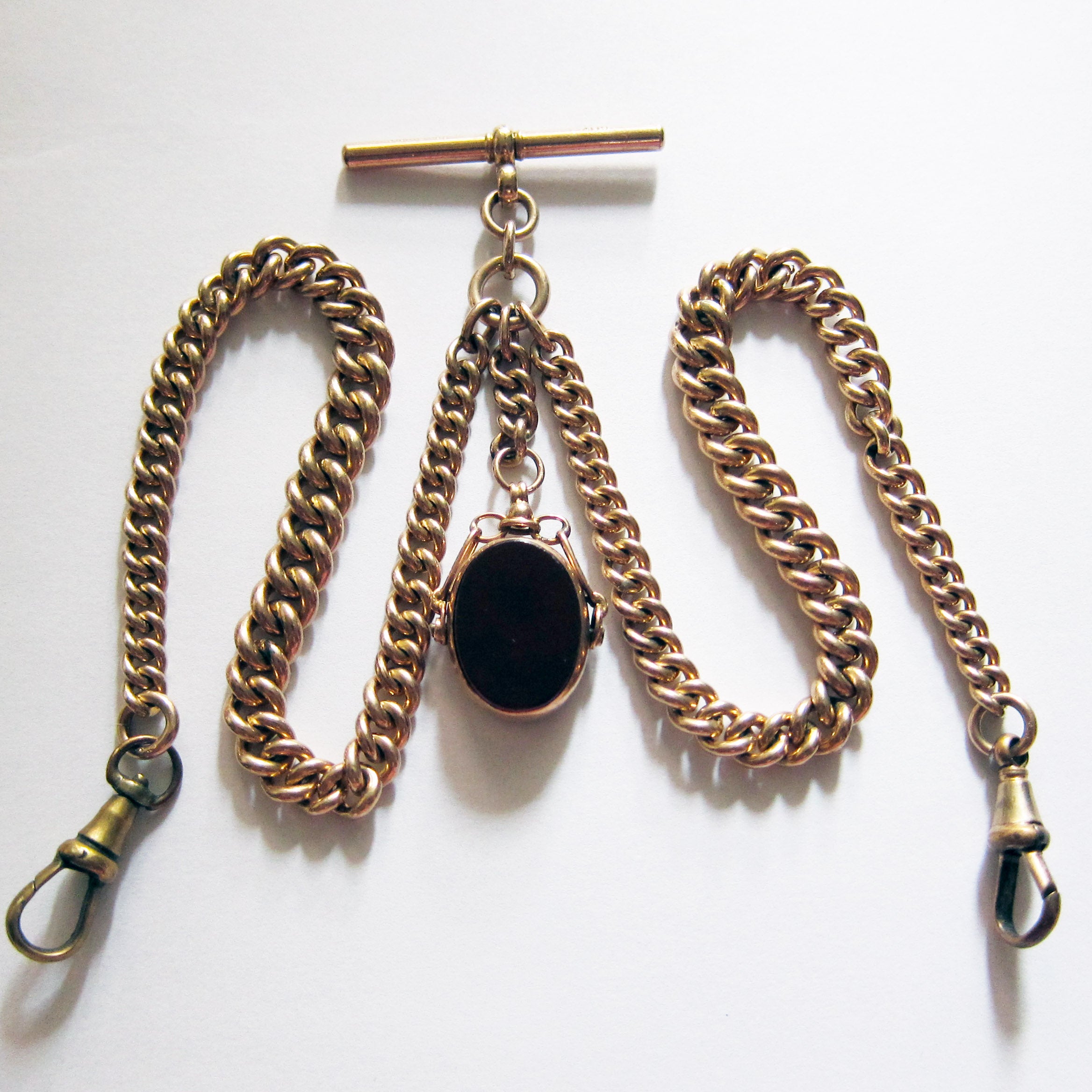The photograph features a predominantly white background, subtly shaded with shadows to create depth. Centrally laid out on this surface is a thick, gold-colored chain, resembling the consistency and structure of a rope. The chain is comprised of multiple interlinked loops, adorned with clasps at both ends, suggesting it could be fastened or secured to other objects. The chain forms a serpentine, almost cursive 'W' shape, though some may interpret this as an 'M'. At the top center of this shape, a series of connected rings, progressing from larger to smaller, culminate in a dull yellow horizontal bar, slightly leaning to the left, which is pivotal in anchoring the chain’s layout. Below this assembly, descending from the middle of the chain, hangs a solid black oval pendant, devoid of any markings. The combined elements and layout suggest a piece of jewelry meticulously presented against the clean, white backdrop.